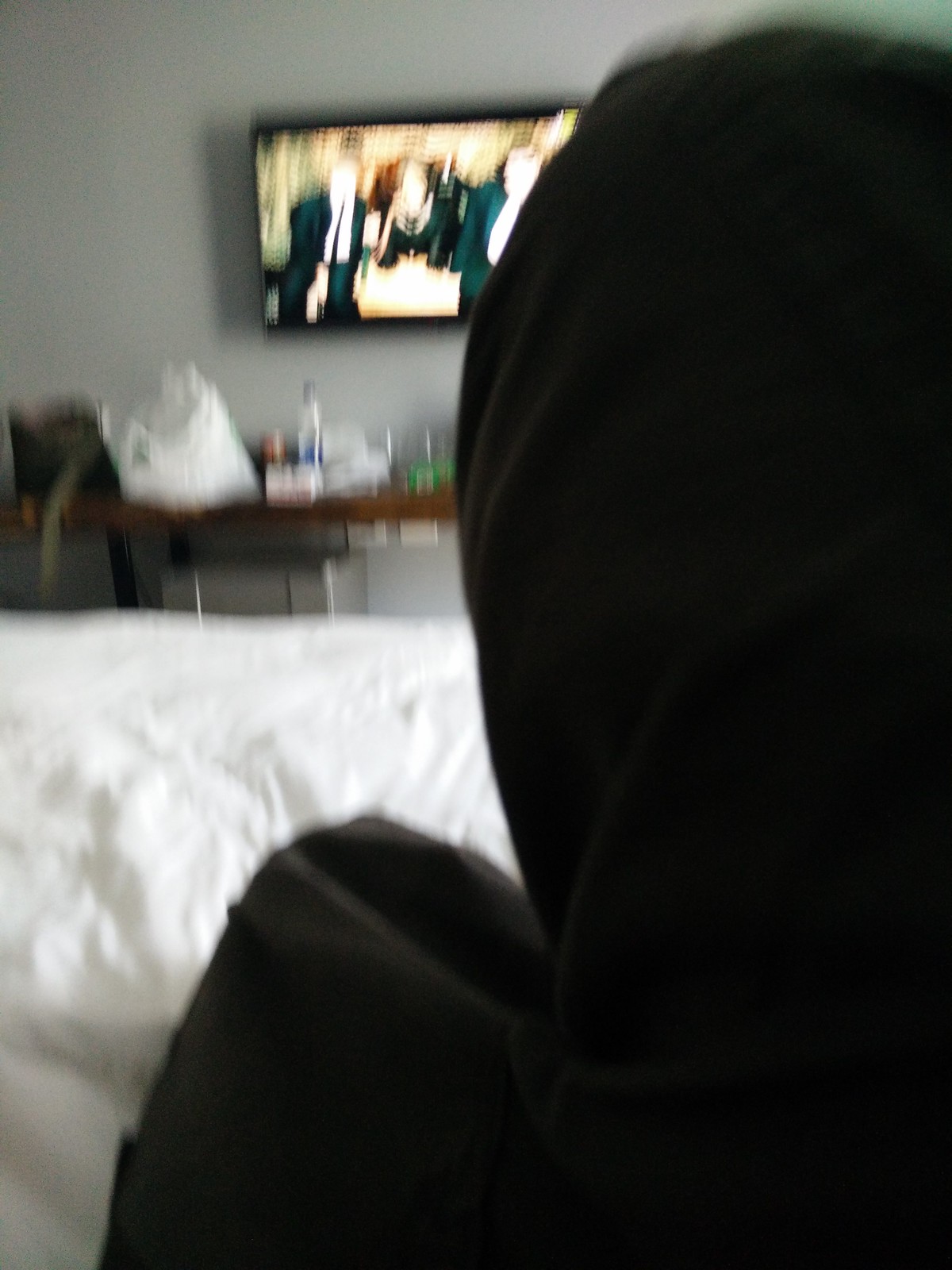This photograph captures a blurry view from someone lying on a bed in a hotel room, with their legs folded and visible, dressed in black pants. The medium-gray wall in front of them has a flat-screen television mounted on it, playing a show featuring two men in suits, possibly both wearing ties, flanking a woman in a black top. Below the television, a wooden desk holds several indistinct items—a white plastic shopping bag, a tall clear bottle, a few drinking glasses, a brown can, and a green package. Partially in the frame, the back of a person can be seen, possibly in a dark green garment and hooded head covering, watching the television.